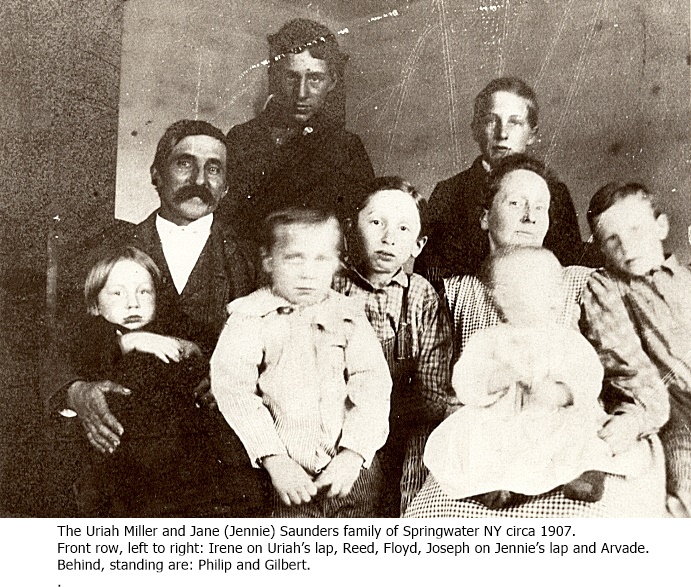The image is a black-and-white photograph of the Uriah Miller and Jane "Jenny" Saunders family from Springwater, New York, circa 1907. The photo captures the entire family with a caption providing their names and positions. In the front row, from left to right, there is Irene sitting on Uriah's lap, Reed, Floyd, Joseph on Jenny's lap, and Arvid. Standing behind them are Philip and Gilbert. Uriah and one of the young boys in the front row wear black suits, while another boy is dressed in a white jacket and one in a checkered shirt with overalls. Jenny sports a checkered apron and holds a baby in a white dress, whose face is slightly blurry due to the long exposure time, as are a couple of other family members’ faces. The photograph itself shows signs of age with noticeable dust, scratches, and possibly reflections from being scanned. To the left in the background, there is a dark door with a visible handle, and some black spots can be seen on the right side of the wall. Overall, the family members are all looking at the camera, evoking a sense of solemn presence characteristic of early 20th-century photography.